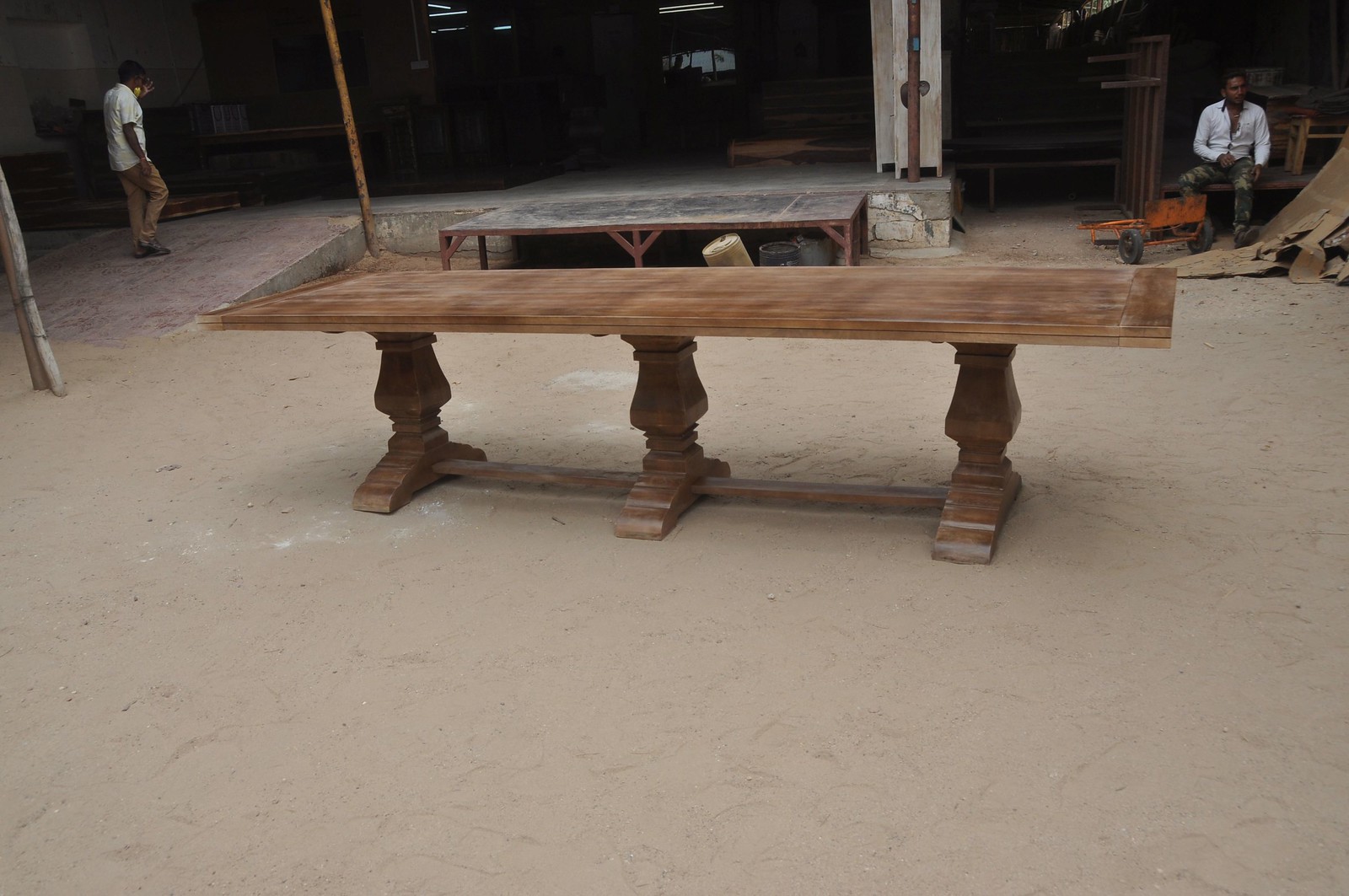This photograph captures an outdoor workspace that appears to be part of a furniture factory or carpentry shop, possibly in another country. The ground is sandy, reddish clay or dusty dirt, giving the entire scene a rugged appearance. Dominating the foreground is a large, long rectangular wooden table. The table is a light rustic brown and features three heavy, circular pedestals as legs, each connected by wooden braces for added stability. Though dusty and covered in dirt, the craftsmanship of the table is evident, and it appears to be a piece that will look striking once cleaned and polished.

In the background of the image, two dark-skinned men, possibly of Mexican descent, can be seen. One man, wearing a white shirt and camel pants, is seated on a bench, while the other, dressed similarly in a white shirt and brown pants, is walking up a ramp that leads to a concrete floor. This ramp is part of the warehouse or industrial area that dominates the upper part of the image. The warehouse itself is open-walled, revealing various elements such as workstations, wheelbarrows, and a rusted platform. The lighting is dim, but some artificial lights are visible on the ceiling, enhancing the industrial atmosphere.

Additional elements in the scene include a small red wagon or dolly near the seated man and a pile of broken plywood or cardboard. Another table with a metal frame is positioned further back, contributing to the sense of an active workspace amidst the gritty environment.